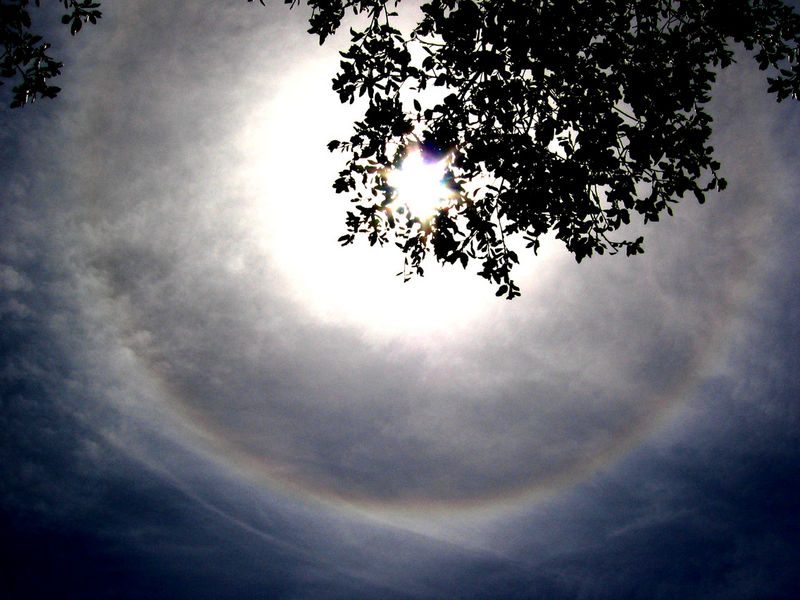This vibrant color photograph captures a striking celestial phenomenon in the daytime sky. The image, taken from the ground, shows the Sun shining brightly through the wispy, milky clouds above. Tree branches and leaves, in silhouette, overhang and partially obscure the luminous orb of the Sun. The sky varies from patches of darker blue to lighter hues, painting a picturesque backdrop. Surrounding the Sun is an impressive halo, reminiscent of a rainbow, encircling the clouds in geometric patterns. This halo effect creates a mesmerizing and almost eclipse-like appearance, with beams of sunlight peeking through the gaps in the leaves, enhancing the ethereal quality of the scene. The intricate interplay of light and shadow framed by the natural elements of the tree and sky makes for a compelling and beautiful photograph.